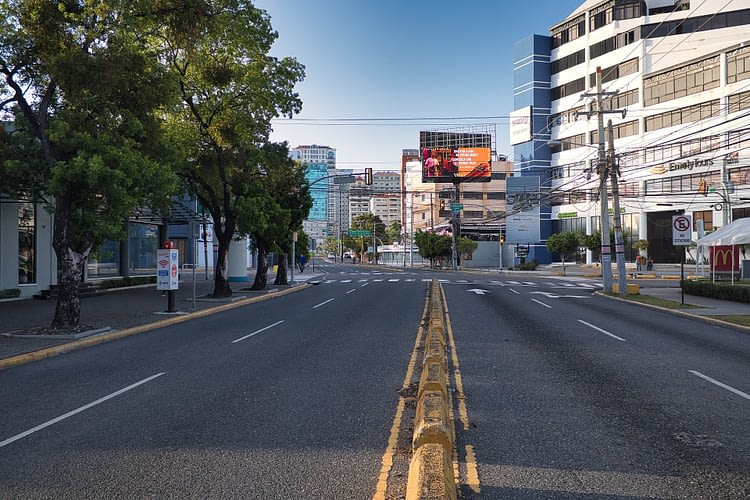The photograph captures a dynamic downtown city street, taken from the middle of an intersection devoid of traffic, suggesting a typically busy area. The street consists of two lanes in each direction, split by a continuous line of yellow concrete dividers reminiscent of parking lot barriers. Surrounding the intersection are diverse elements: lush green trees line the sidewalk, and a mixture of small and large buildings create an urban landscape, their facades featuring a spectrum of colors including white, blue, and hints of orange seen in a banner. Overhead, power lines bisect the sky, hinting at the practical necessities of city life. Street signs, though indistinct, appear to be in English, amidst a plethora of street posters and a prominent billboard on the left. To the right, a McDonald's sign punctuates the urban scene, affirming a familiar commercial presence. The vantage point of the photo clearly places the viewer at street level, emphasizing the straightforward and bustling nature of this city setting.